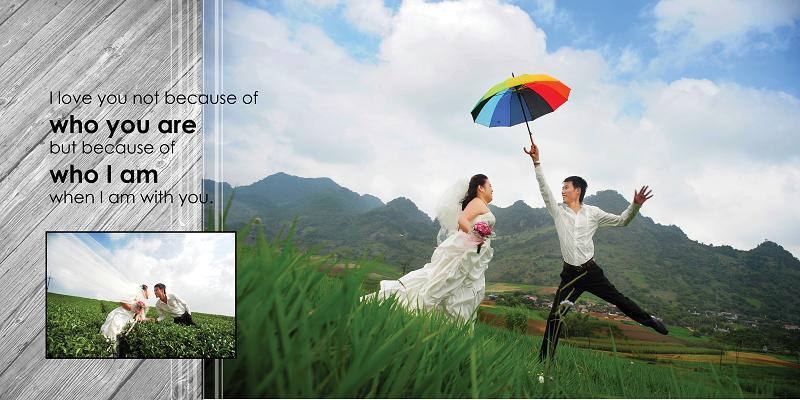This vibrant color photograph captures an outdoor wedding scene, featuring an Asian bride and groom against a breathtaking backdrop of mountains and an expansive sky filled with scattered white clouds. The bride, adorned in a traditional sleeveless white wedding gown and a veil, is holding a bouquet of pink flowers while standing on lush green grass. She faces the groom, who is energetically jumping in the air, dressed in black dress slacks and a white long-sleeved dress shirt. His right arm is extended upwards, holding a rainbow-colored umbrella, and his legs are spread wide in mid-air, with his left leg higher than his right.

The composition is dynamic, with the camera positioned at ground level, capturing details of the close-up grass blades. A grayish-green border on the left side houses black text that reads: "I love you not because of who you are, but because of who I am when I am with you." Additionally, there is a smaller inset within this border showing another image of the couple kissing in a field. The weather appears comfortably warm, with an overcast sky diffusing the light evenly across the scene. In the distance, some buildings are visible at the base of the mountains, suggesting an idyllic yet possibly familiar setting for the couple.